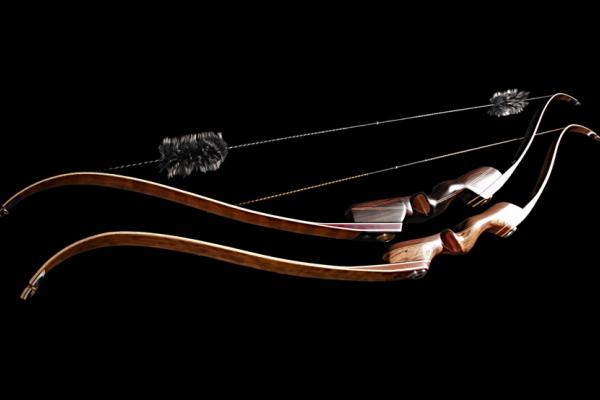This photograph captures two highly polished, decorative recurve bows, crafted from wood and contrasting in color. They are arranged one atop the other against a completely black background, enhancing their bright, shiny appearance. The top bow features distinctive black and gray fuzzy tufts at both ends of its tightly strung string. Both bows showcase intricate craftsmanship, with handles stained in red and tan tones, giving them a traditional, almost antique look. Despite their decorative elegance, the sturdy build suggests functional capability, though their pristine condition hints at their role as more ornamental than utilitarian.